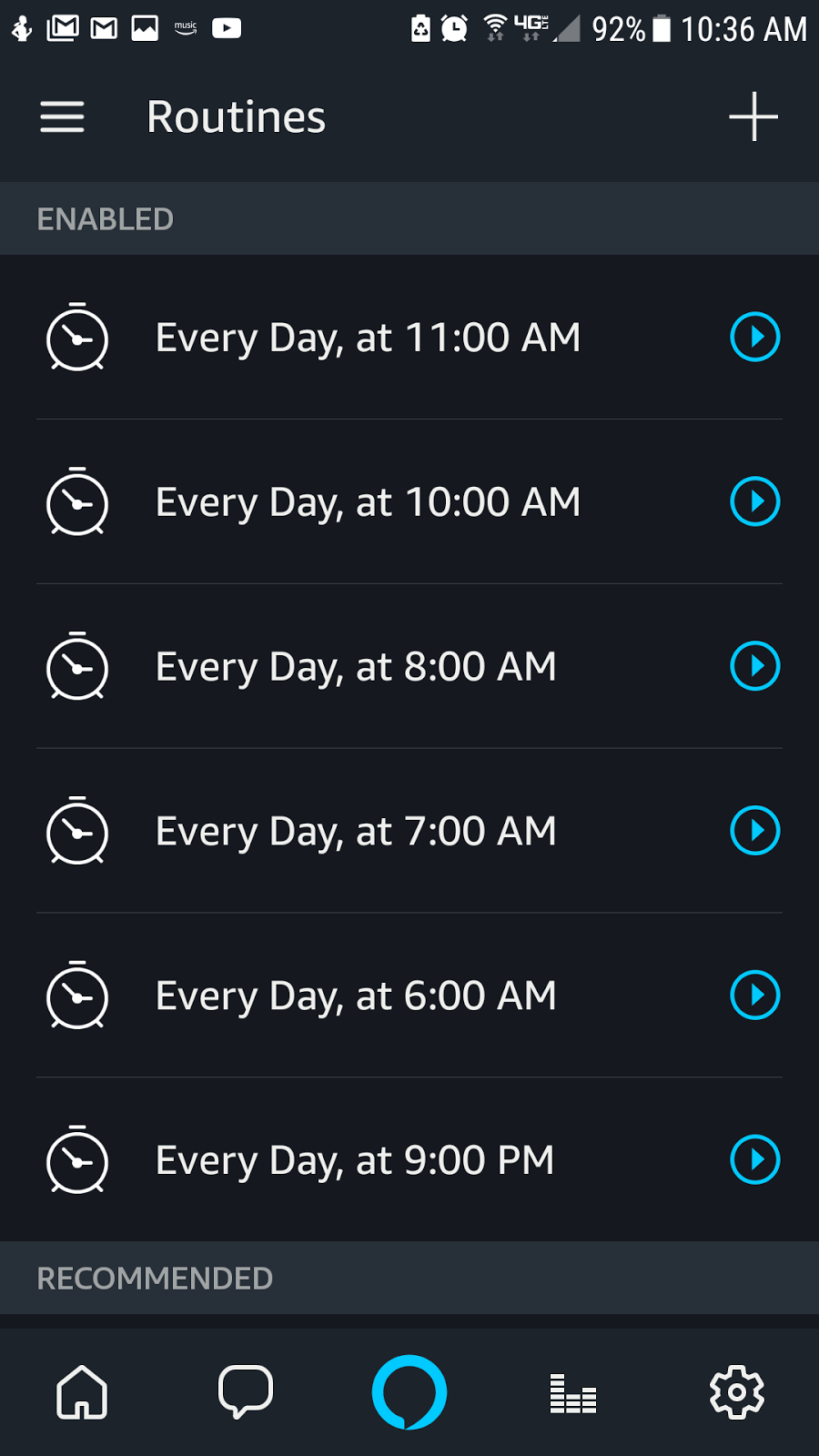A detailed screenshot of a smartphone's home screen taken at 10:36 a.m. is displayed. The battery is at 92% and the device is connected to a 4G network with poor signal strength, showing almost no bars. However, the Wi-Fi connection is strong with full bars. Notifications from several apps are visible, including Gmail, Amazon Music, and YouTube.

In the upper section of the screen, there's an alarm clock set, and various menu options are displayed. A three-line menu icon indicates a drop-down menu, followed by the word "Routines" and a plus sign option for adding new routines. Below, the word "Enabled" is displayed.

The screen lists several daily alarms with identical blue play buttons on the right side:
- Every day at 11 a.m.
- Every day at 10 a.m.
- Every day at 8 a.m.
- Every day at 7 a.m.
- Every day at 6 a.m.
- Every day at 9 p.m.

The section titled "Recommended" is also noted, although no details are provided about its content.

At the bottom of the screen, there are navigation icons for Home, Messages, a blue circle, and Settings.